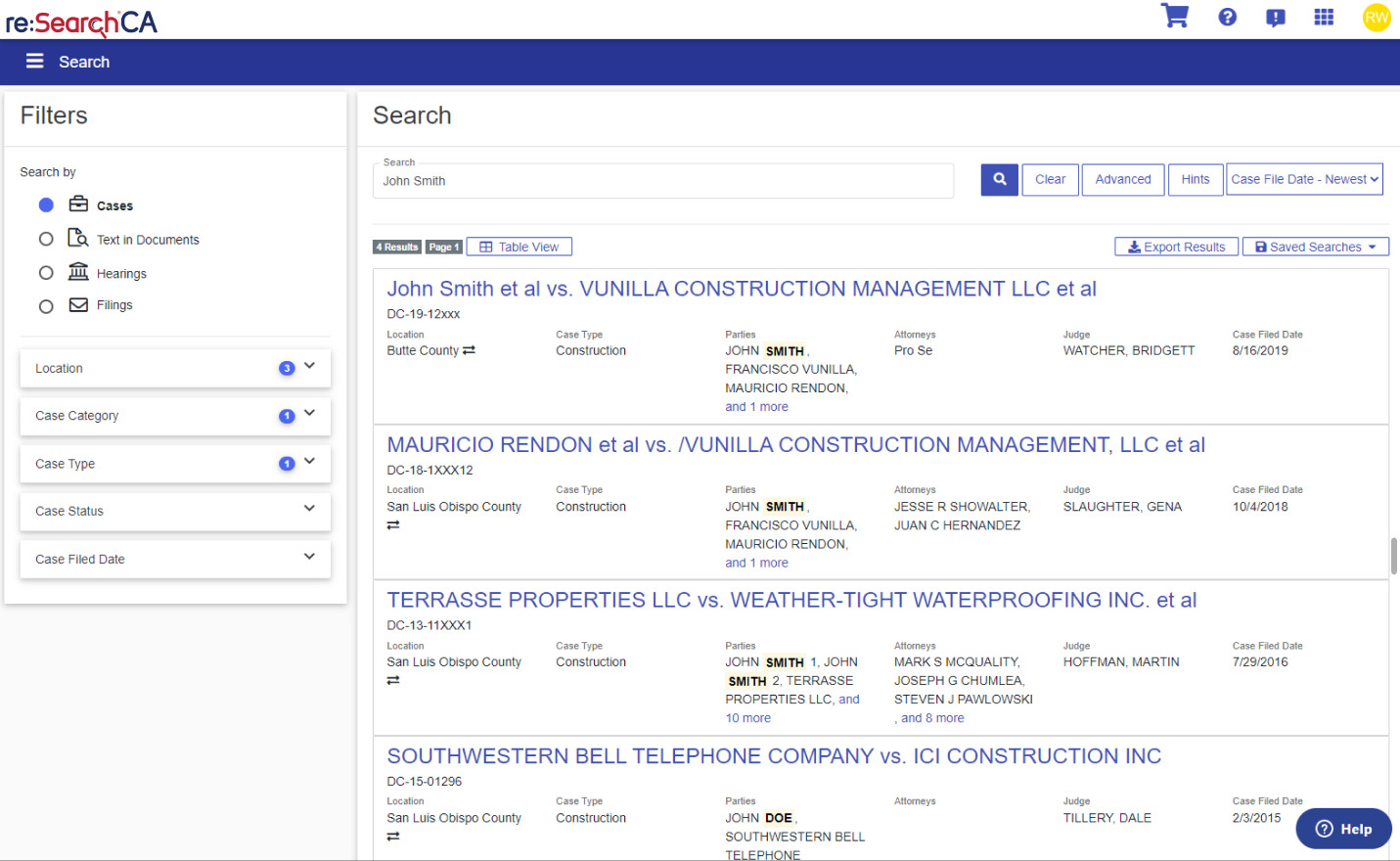This is a desktop screenshot of what appears to be an application, possibly a web-based platform, given the absence of an address bar. The application is titled "reSEARCH CA" with "re" in lowercase and "SEARCH CA" capitalized. On the far right of the white header bar, there are several icons: a dark blue shopping cart, a question mark, an exclamation mark in a text box, a semblance of a keypad, and an RW within a yellow circle.

The interface is divided into two main sections. The left section, occupying about a quarter of the screen, features a navigation menu titled "Filters." This menu allows users to search by:
- **Cases** (represented by a briefcase icon)
- **Text and Documents** (represented by a magnifying glass over a paper icon)
- **Hearings** (represented by a courthouse icon)
- **Filings** (represented by an envelope icon)

Currently, the "Cases" option is highlighted. Below these options, additional filters include:
- **Location** (with a dropdown indicating 3 selections available)
- **Case Category 1**
- **Case Type 1**
- **Case Status**
- **Case File Date**

The right section, covering the main part of the screen, displays search results for "John Smith." At the top of this section, there's a blue search button (magnifying glass icon) and white boxes labeled "Clear," "Advanced," and "Hints." Additional filter options include "Case File Date: Newest."

Following this, the results area indicates "4 results, page 1." It also offers options to switch to "Table View," export results (down arrow into a box icon), and save searches (blue floppy disk icon).

The detailed case results are displayed as follows:

1. **John Smith et al. vs. Bunilla Construction Management LLC et al.**
   - **Docket Number:** DC 1912 (Partially redacted)
   - **Location:** Buck County
   - **Case Type:** Construction
   - **Parties:** John Smith, Francisco Bunilla, Mauricio Rinden, and one more.
   - **Attorneys:** Pro Se
   - **Judge:** Watcher Bridget
   - **Case Filed Date:** August 16, 2019

2. **Mauricio Rinden et al. vs. Bunilla Construction Management LLC et al.**
   - **Docket Number:** DC 1818 1xxx12
   - **Location:** San Luis Obispo County
   - **Case Type:** Construction
   - **Parties:** John Smith, Francisco Bunilla, Mauricio Rinden, and one more.
   - **Attorneys:** Jesse R. Showalter, Juan C. Hernandez
   - **Judge:** Gina Slaughter
   - **Case Filed Date:** October 4, 2018

3. **Taurasi Properties LLC vs. Weathertight Waterproofing Inc. et al.**
   - **Docket Number:** DC 13-11xx1
   - **Location:** San Luis Obispo County
   - **Case Type:** Construction
   - **Parties:** John Smith, Taurasi Properties LLC, and 10 more.
   - **Attorneys:** Mark S. McQuality, Joseph G. Chumlea, Steven J. Pawlowski, and eight more.
   - **Judge:** Martin Hoffman
   - **Case Filed Date:** July 29, 2016

4. **Southwestern Bell Telephone Company vs. ICI Construction Inc.**
   - **Docket Number:** DC 1501296
   - **Location:** San Luis Obispo County
   - **Case Type:** Construction
   - **Parties:** John Doe, Southwestern Bell Telephone
   - **Attorneys:** None listed
   - **Judge:** Dale Tillery
   - **Case Filed Date:** February 3, 2015

This interface likely serves as a search tool for a database of judicial cases in California.